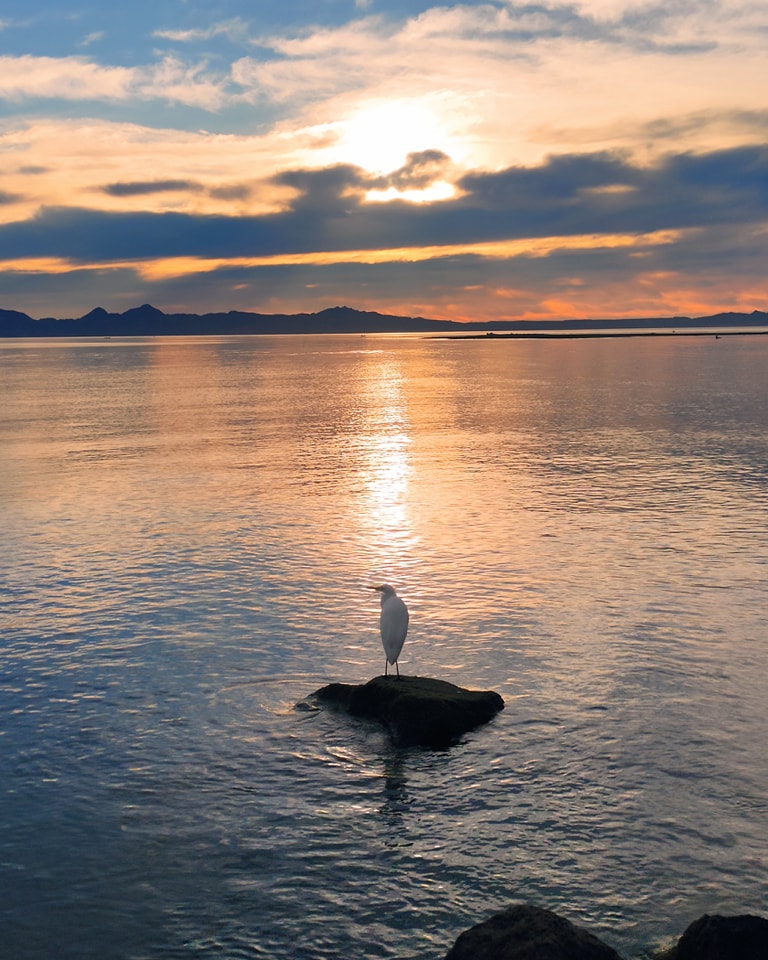The image captures a breathtaking sunset over a serene body of water, possibly a lake or bay, with a shimmering surface reflecting the vibrant colors of the sky. The sun, partially obscured by dark clouds, casts a beautiful gradient from yellow to orange as it descends toward the horizon. In the foreground, a black rock juts out from the water, adorned by a solitary white bird with a yellowish beak, resembling an egret. The bird stands poised, gazing towards the left. The background features hilly or mountainous terrain with a hint of trees, further enhancing the natural beauty of the scene. A sliver of land extends into the calm, bluish water, which transitions to shimmering reds and whites closer to the horizon, reflecting the brilliant sunset. A distant landmass and what appears to be a wharf add depth to the tranquil setting, giving a sense of a peaceful evening at a secluded lakeshore or bay.